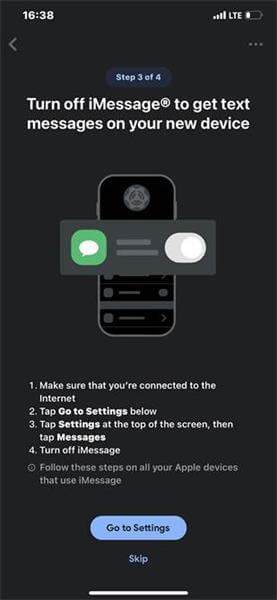A screenshot from a mobile phone with a black background is being displayed. At the top, the time is shown as 16:38, alongside LTE cellular connectivity and a battery icon that is approximately one-fourth full. Moving slightly lower, there is a back arrow on the left and three horizontal white dots on the far right.

Centrally located on the screen is an oval-shaped area displaying the progress "Step 3 of 4" in white text. Below this, it instructs the user to "turn off iMessage to get text messages on your new device," with corresponding visual aids: an image of a phone, a green square featuring a white speech bubble, and a slider currently set to the "on" position.

Further down, the instructions are listed vertically:

1. Make sure that you're connected to the internet.
2. Tap 'Go to Settings' below.
3. Tap 'Settings' at the top of the screen, then tap 'Messages.'
4. Turn off iMessage.

The reminder includes an additional note to perform these steps on all Apple devices using iMessage. At the bottom of the screen, there are options to "Go to Settings" in a blue circle or to "Skip."